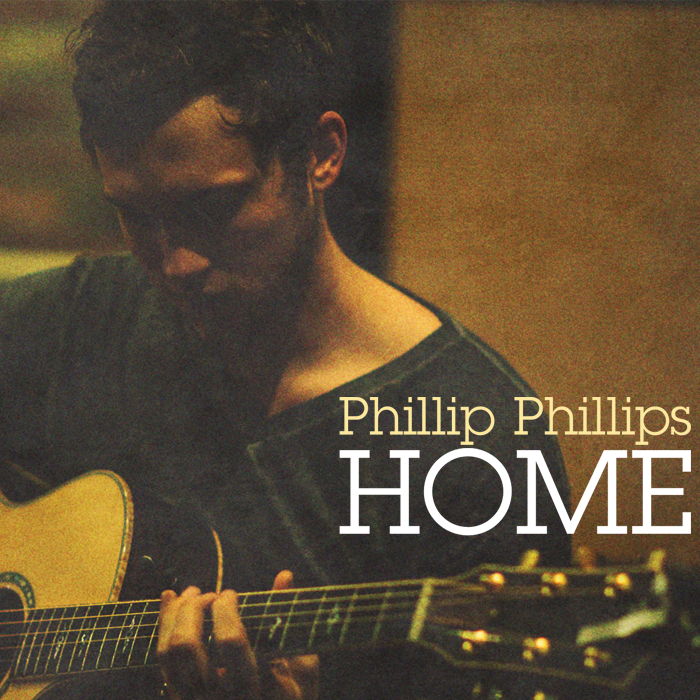The album cover features a grainy image with a brown, shadowy backdrop. On the left side of the picture, a white man with tousled dark hair and a hint of a scruffy beard is seated, visible from his torso up. He is wearing a black or dark blue V-neck T-shirt, and his head is slightly bowed as he focuses on playing an acoustic guitar, with one hand visible on the strings. The guitar has a brown face with a black body. The photo's shadows obscure parts of his face, particularly around his chin, giving him a more mysterious look. On the right side of the cover in yellow font, it reads "Philip Phillips," and beneath it, in larger white font, is the title "Home." The background remains indistinct, with a tan wall and a dark beam partially visible behind the man.